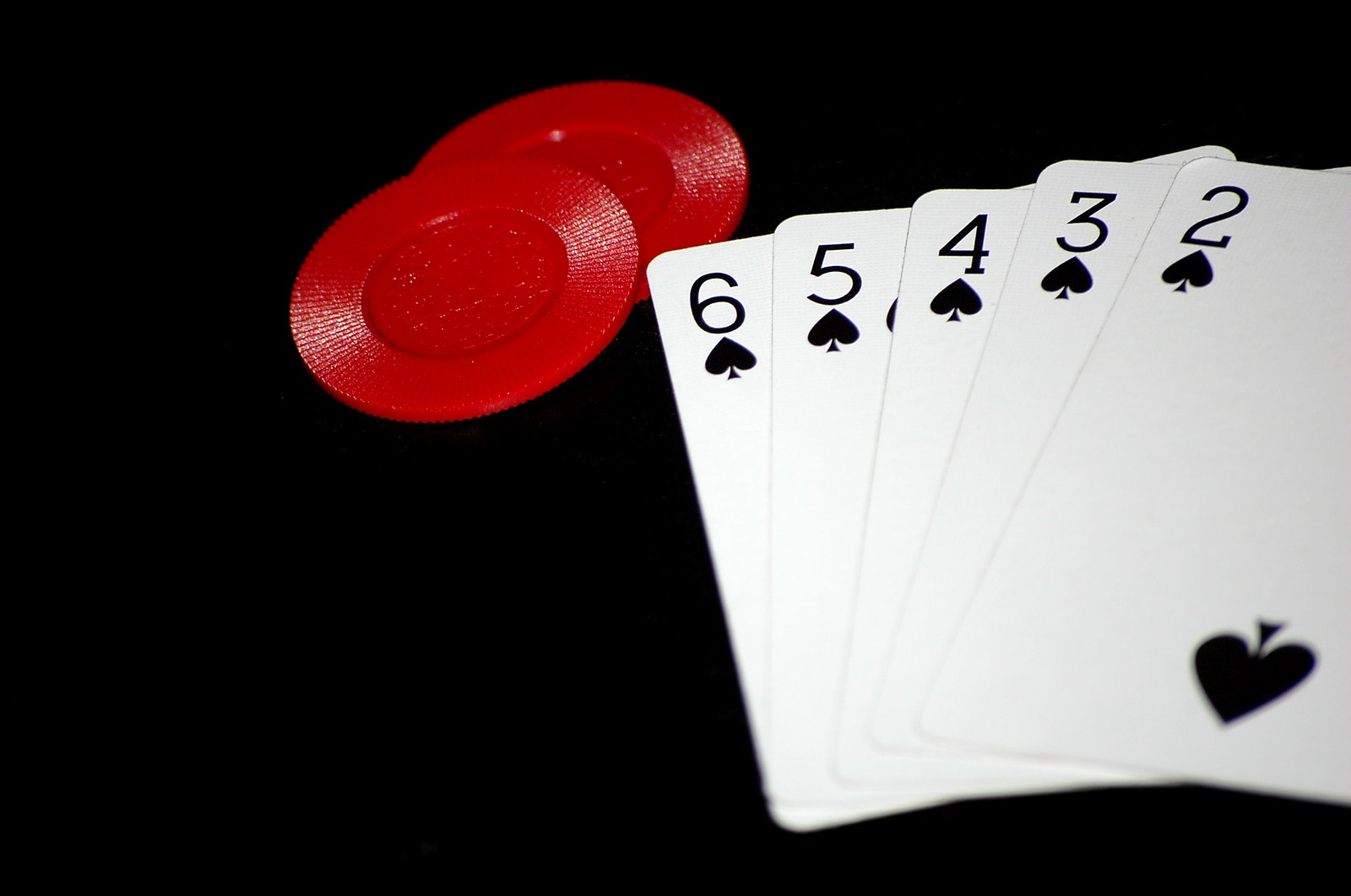This is a meticulously composed photograph featuring five playing cards and two poker chips, set against a uniformly black background. The playing cards are fanned out face-up, displaying a sequential run from the two of spades to the six of spades. The cards are minimalistic in design, with the only notable detail being a single spade symbol on the bottom card. To the left of the cards, two round, shiny red poker chips are positioned, one slightly overlapping the other. The poker chips exhibit ridged edges and a reflective surface that catches the light, hinting at their plastic composition. The stark black background serves to highlight the simplicity and uniformity of the elements in the photograph, ensuring no distractions from the central subjects of cards and chips.